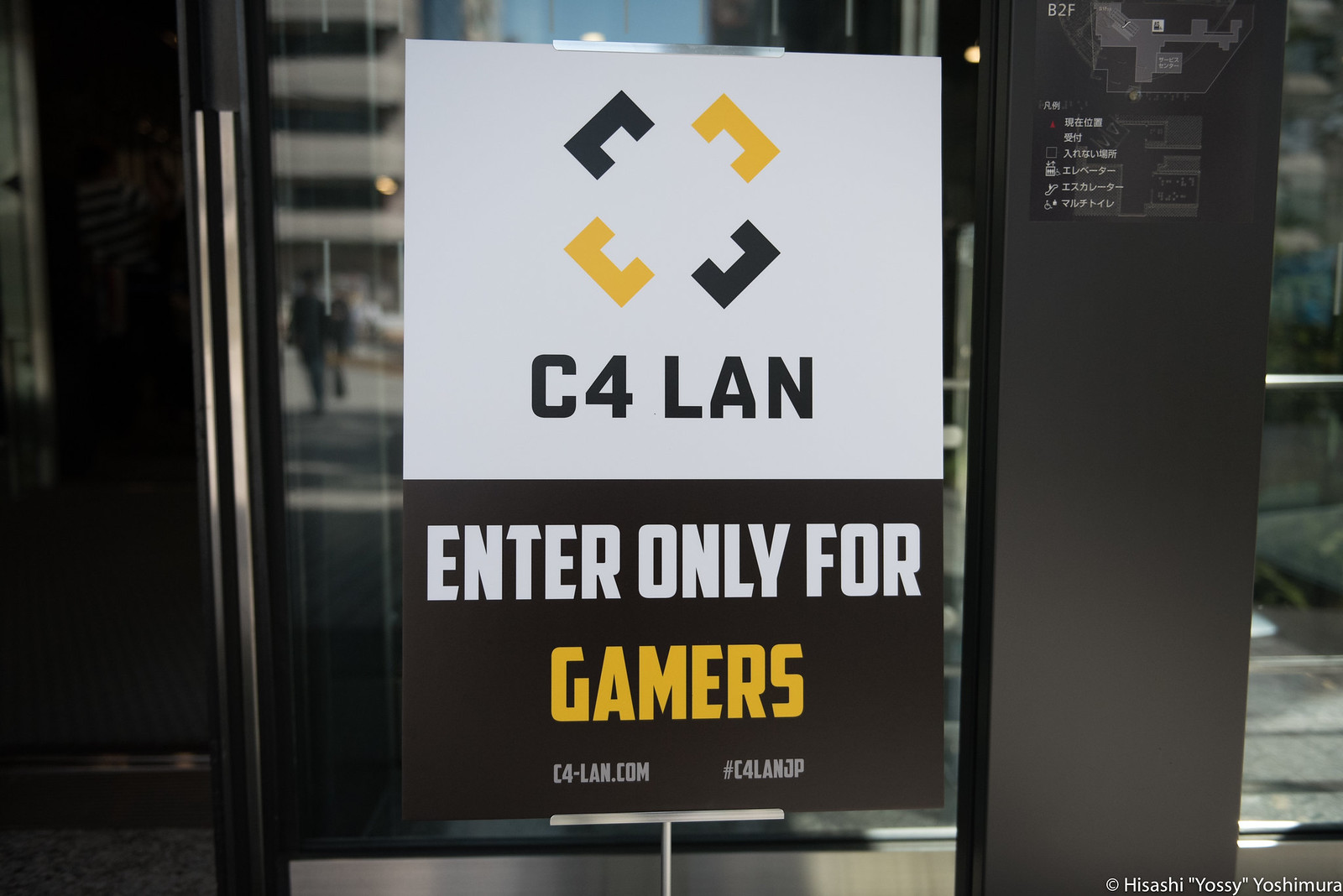The photograph captures an advertisement flyer displayed in front of a glass-paneled door of what appears to be an office or commercial building. The glass doors, which have chrome-colored handles, are accompanied by columns with a dark bronzy color. The advertisement itself is mounted in a shiny metal frame and showcases a distinct logo consisting of four thick square brackets arranged to form an X on a white background. The title "C4 LAN" is prominently featured below the logo in bold black text. The bottom part of the flyer has a dark background with the message "Enter Only For Gamers" written in white text, with "Gamers" highlighted in yellow. At the very bottom of the flyer, there is a website, "c4-lan.com", and a hashtag, "#C4LANJP," suggesting the flyer is related to a Japanese gaming community or event. Additionally, some Japanese characters can be seen near the banner on an adjacent column, reinforcing the clue that this is set in Japan.